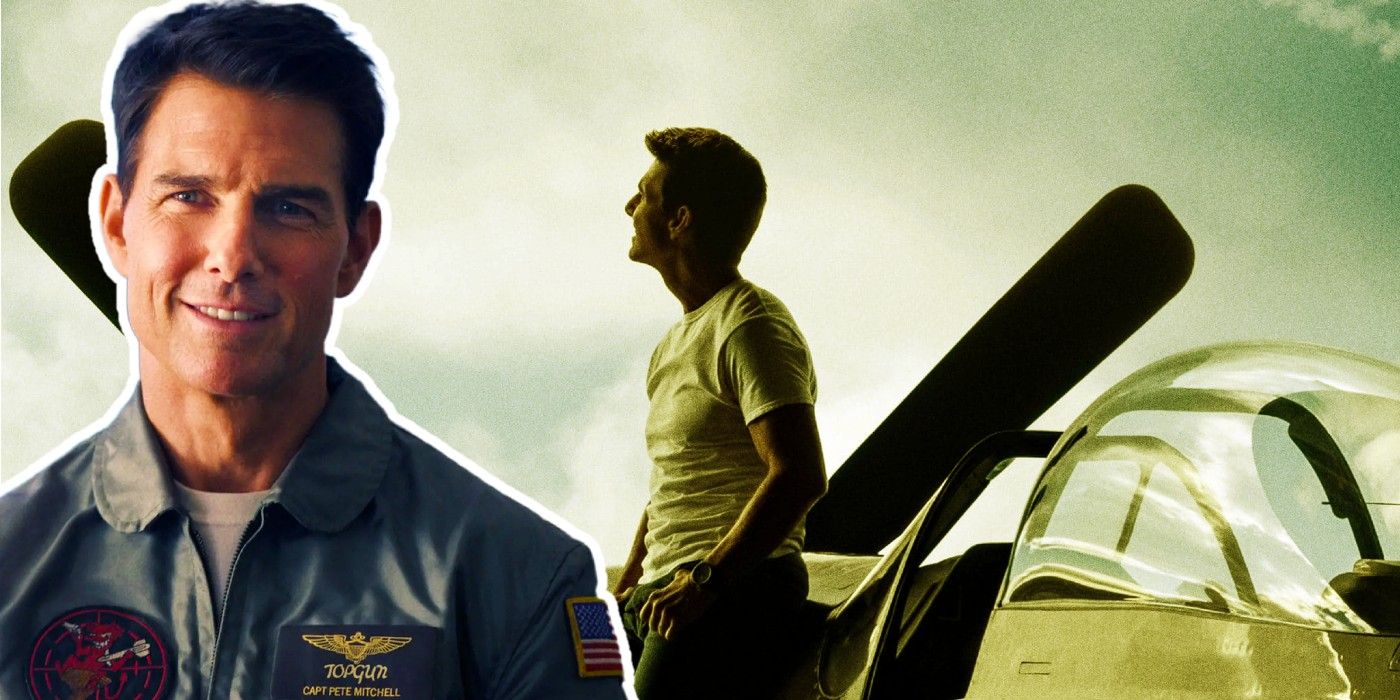The photograph is a detailed color montage from the movie "Top Gun," prominently featuring two distinct images of Tom Cruise. On the left side, Tom Cruise, the older version, stands in his iconic Top Gun uniform - a fighter suit adorned with an American flag patch on his left shoulder. His aviator jacket is decorated with a variety of patches, including a prominent yellow eagle on the right chest and a black circle with red embroidery on the left. He is smiling directly at the camera against a backdrop of a blue and white sky. To the right, another image captures Tom Cruise in a casual outfit consisting of a white t-shirt and jeans, with a watch on his left wrist. He is looking upwards, seemingly into the sky, while leaning on the canopy of a fighter jet with its gleaming windshield visible. The background of this section also features white clouds against a serene blue sky.